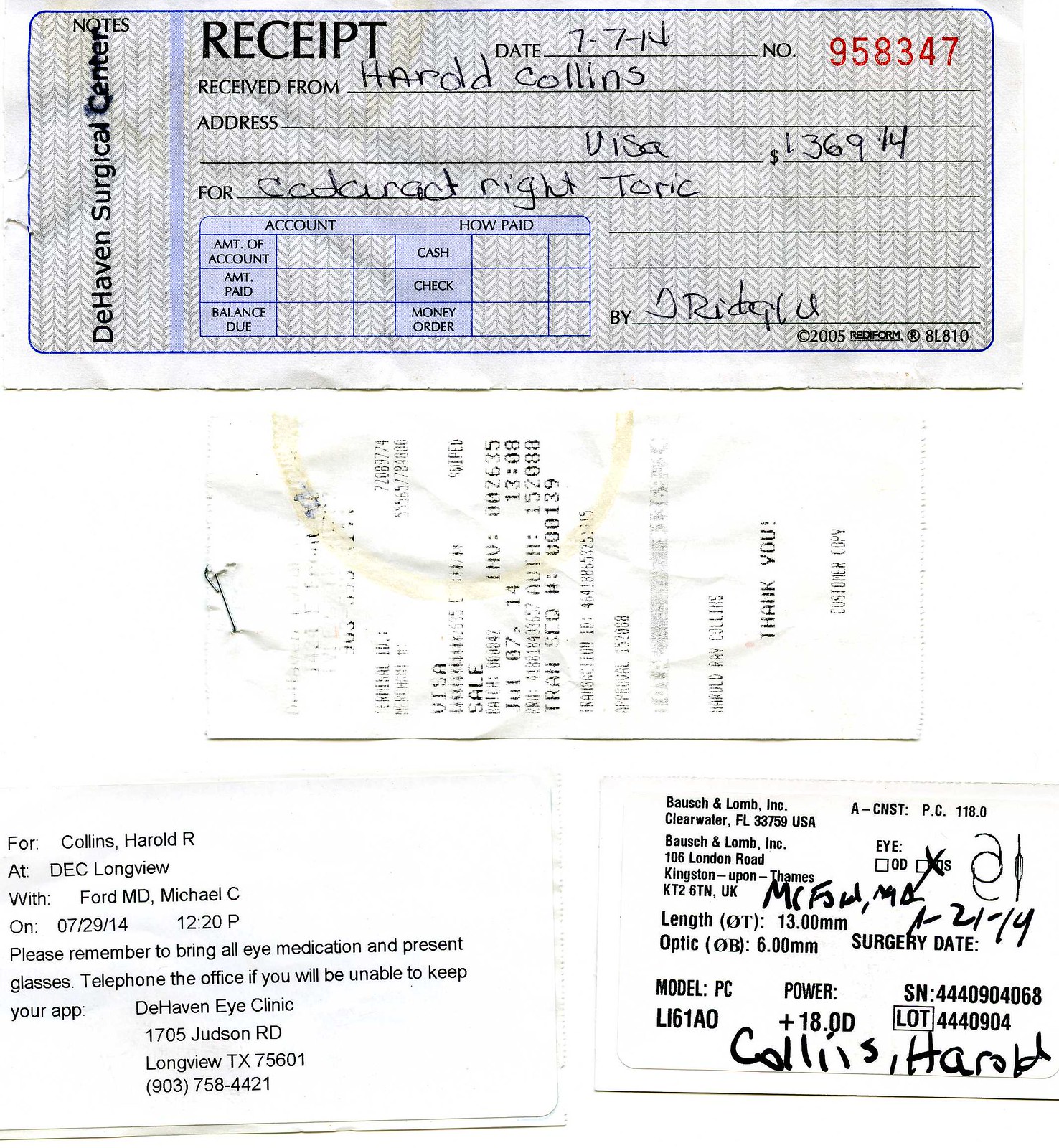This detailed photograph displays a collection of scanned and photographed receipts, appearing to be part of a record-keeping system. The top section of the image prominently features a detailed receipt from Dehaven Surgical Center, dated 07/07/14, with a reference number 958347. This receipt totals $1,369.14 for a cataract right toric procedure. Below this, a faded receipt, likely from a gas station, is partially visible but unclear. 

In the bottom left-hand corner, there is a more legible receipt associated with Collins Herald, mentioning a December appointment at Longview, and instructions to bring all eye medication and present glasses along with contact information for Dehaven Eye Clinic. The bottom right-hand corner showcases a receipt from Bausch & Lomb Incorporated, Clearwater, Florida, 33759. 

Overall, the image consolidates various receipts related to medical expenses and prescriptions for glasses, indicating a meticulous effort in documenting and organizing these records.